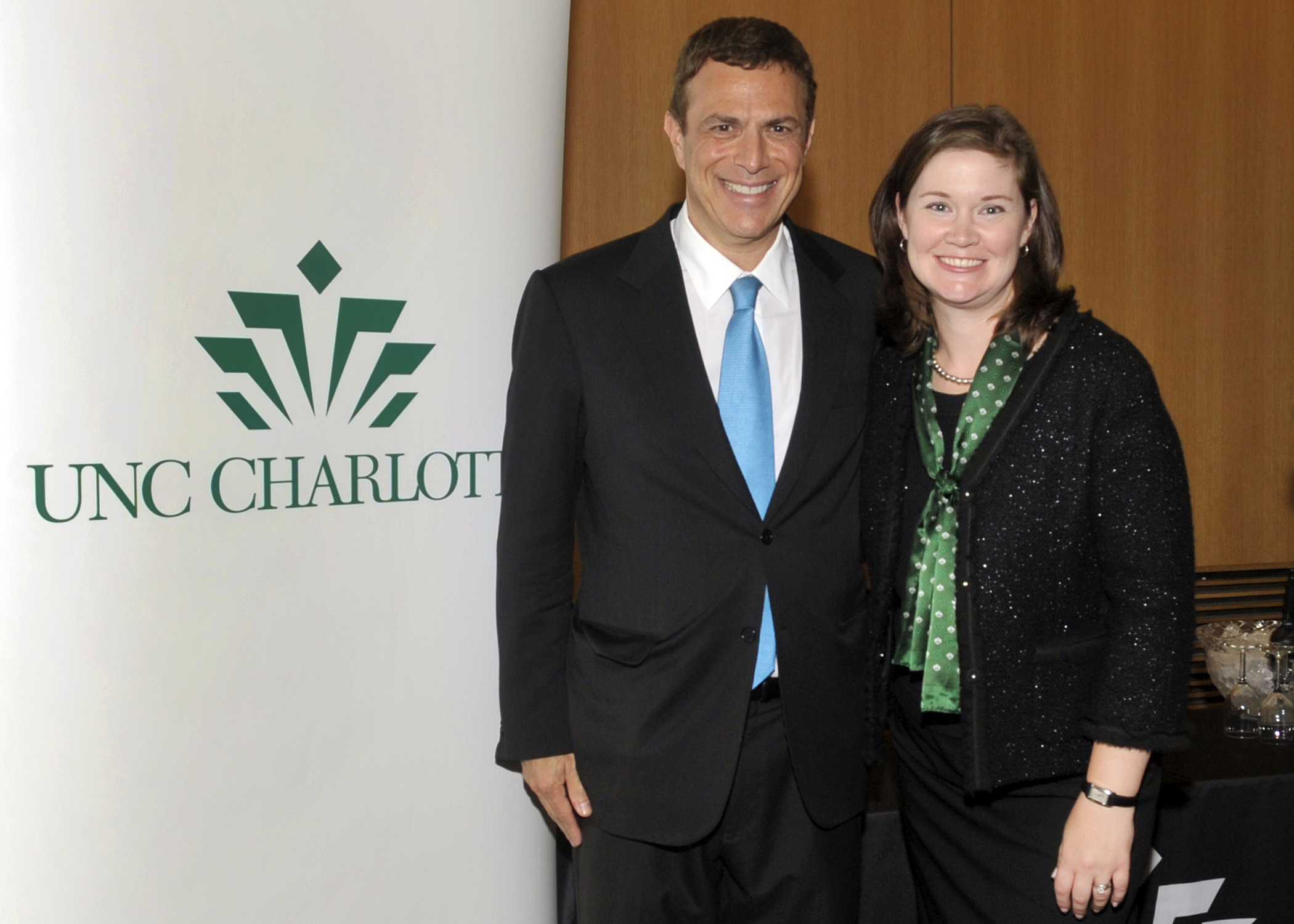The image captures a well-organized scene divided into two distinct sections. In the background, the left side features a white wall adorned with green text spelling "UNC Charlotte," though some of the letters are partially cut off. Above the text is a logo depicting a figure with outstretched arms in a graduation gown, their head bowed, making the cap appear diamond-shaped.

Centered in the frame, two individuals are smiling directly at the camera, suggesting a comfortable indoor setting, likely within a college during daytime. The man on the left side of the image wears a dark suit with a white shirt and a light blue tie. He has dark hair and eyes, a cheerful expression, and his right arm rests by his side, while his left arm is obscured by the woman next to him. The woman, standing very close to the man, has shoulder-length brown hair and is wearing a black sparkly top, a green polka-dotted scarf tied around her neck, a black shell underneath, and a black skirt. She also sports a black watch on her right wrist. Her right arm hangs in front, disappearing behind the man.

Adjacent to the white wall and text, the upper right corner of the image includes a brown wooden cabinet, adding depth and context to the setting. The overall composition and detailed wardrobe and positioning of the individuals make the scene appear formal and collegiate.